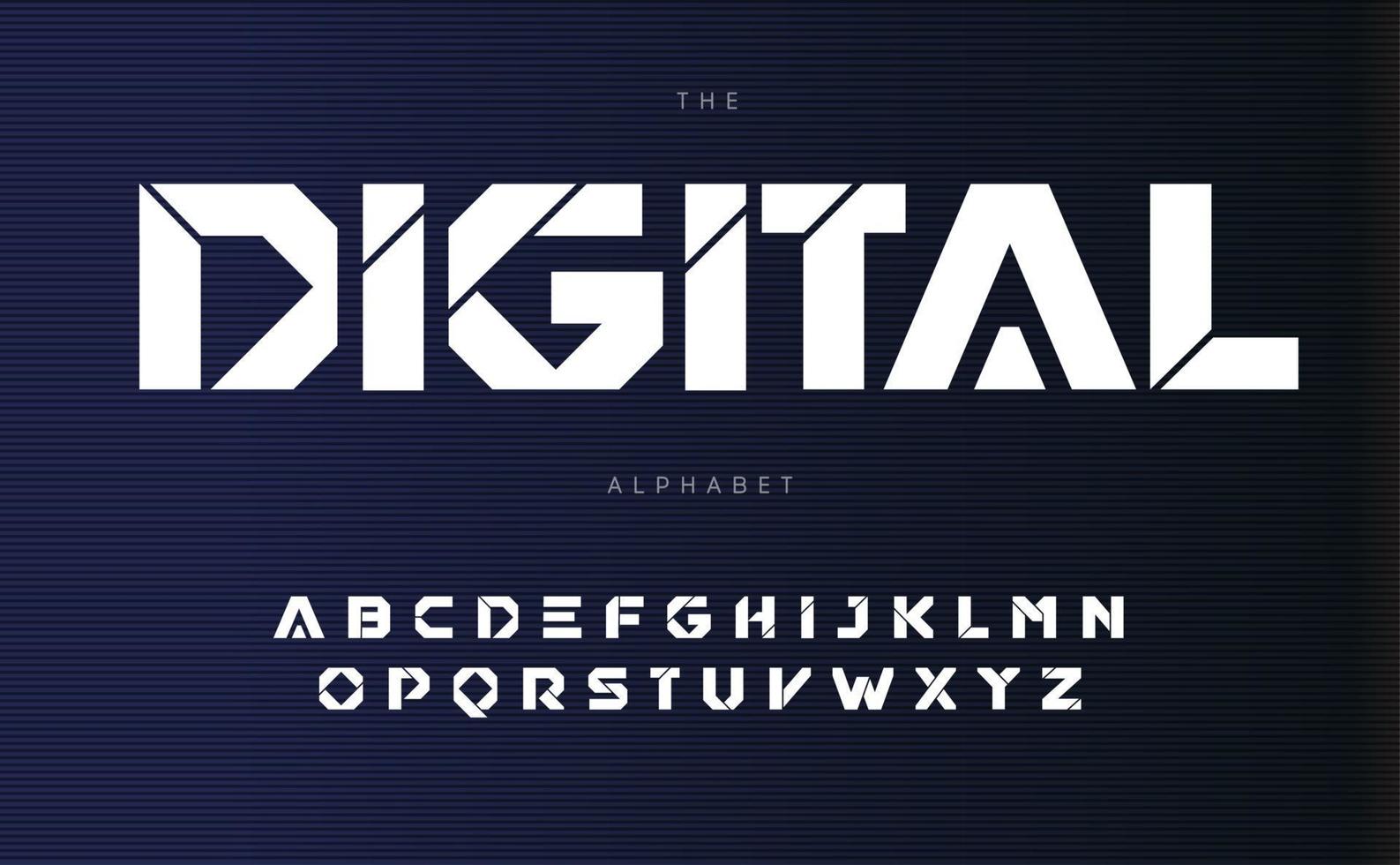The image features a dark blue background that fades to nearly black on the right, with subtle horizontal lines across it. At the top, in small white sans-serif letters, it says "THE," followed by the word "DIGITAL" in larger, blocky, digital-style font with straight and slightly curved lines forming each letter. Beneath this, in small white sans-serif letters, it says "ALPHABET." Below these headings, the alphabet is displayed in uppercase white letters, arranged in two rows: the first row from A to M and the second row from N to Z. The words "DIGITAL" and the alphabet have a bold, digital font style, creating a contrast with the lighter white sans-serif fonts of "THE" and "ALPHABET." The overall design is clean, with no other text or objects in the image, and it maintains a high-quality, focused appearance.